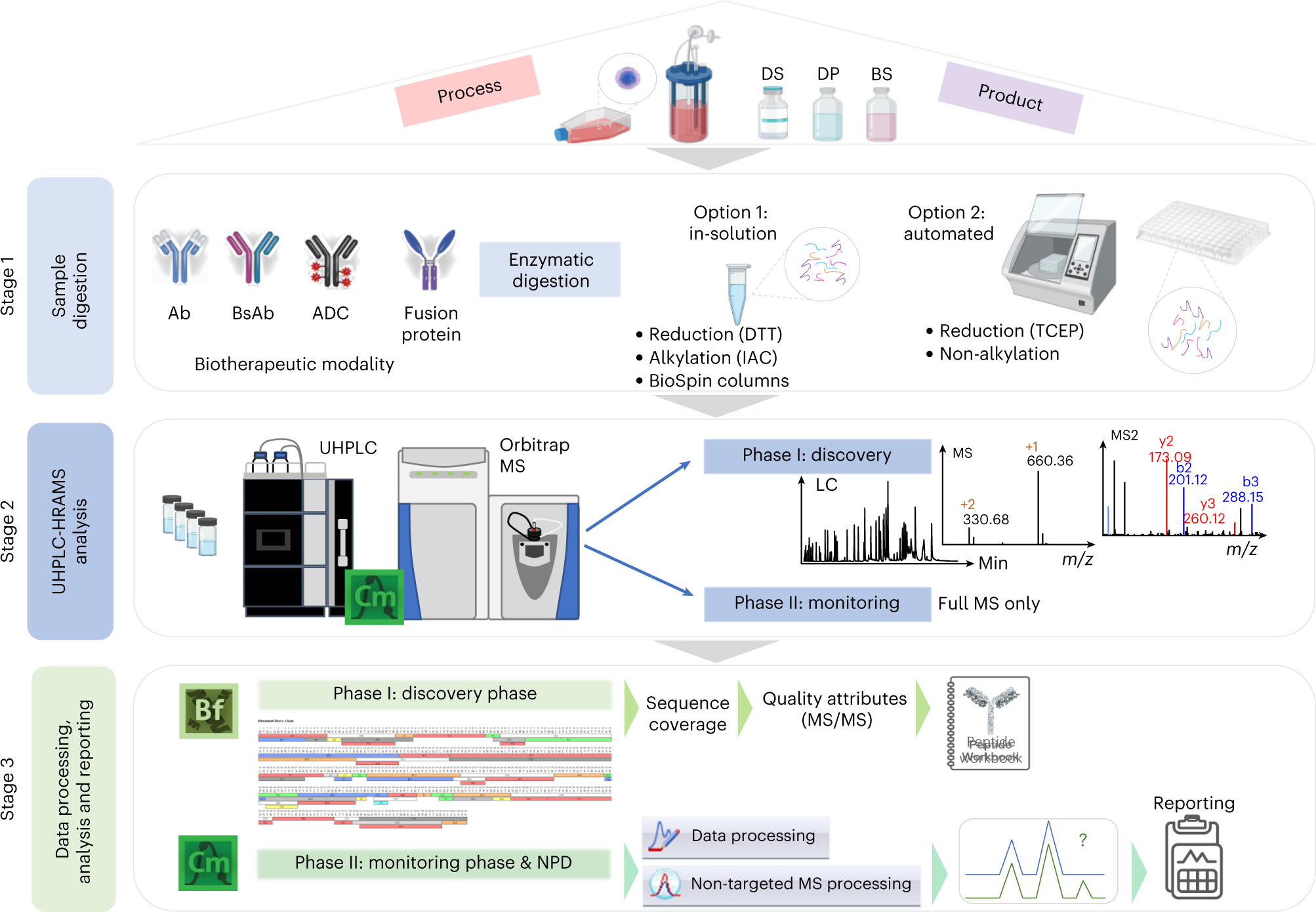This image is an elaborate infographic that outlines a multi-stage scientific procedure. It features a white background with several colored sections and detailed texts. At the top, there are two primary rectangles—one pink labeled "Process" and another also pink labeled "Product." Below these, there are images of bottles labeled "DS," "DP," and "BS," arranged under the text "DSDPBS."

Moving down, the infographic is divided into three stages:

- **Stage One: Sample Digestion** - Displayed in a lavender-colored box, it includes icons denoting "ABBSABADC fusion protein" and mentions "enzymatic digestion." The stage details biotherapeutic modalities, including options for reduction, alkylation, and biospin columns, along with non-alkylation.

- **Stage Two:** Accompanied by another lavender box filled with numbers and letters, this stage is situated next to objects resembling a black and a gray cabinet with wires. Blue arrows link this stage to "Phase One Discovery" and "Phase Two Monitoring."

- **Stage Three: Data Processing Analysis and Reporting** - A green rectangle signifies this stage, accompanied by various icons. It emphasizes the steps of data processing, sequence coverage, and quality attributes.

The infographic is rich in colors like blues, greens, grays, and light purple, and is packed with detailed icons and arrows guiding through the procedural flows, emphasizing phases of discovery and monitoring throughout the scientific process.